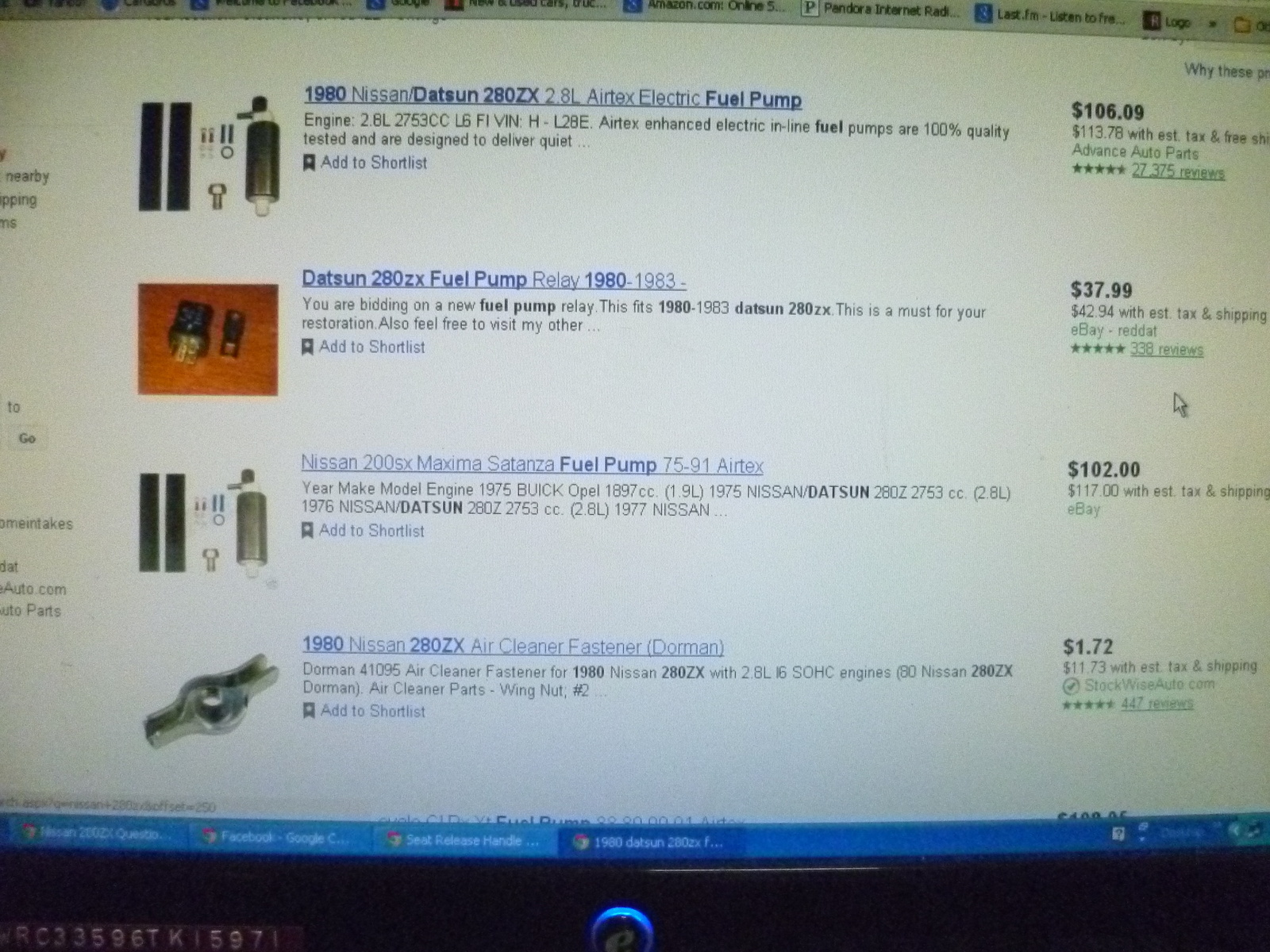A computer monitor displaying an online marketplace page with multiple open tabs at the top. The main focus of the screen is on a specific item listing for a 1980 Nissan Datsun 280ZX 2.8L electric fuel pump. The listing showcases images of the metal fuel pump and includes detailed descriptions. One section of the text reads: "Enhanced electric inline fuel pumps are 100% quality tested and are designed to deliver quiet performance." Another part of the listing highlights a fuel pump relay, stating: "Datsun 280ZX fuel pump relay 1980-1983. You are bidding on a new fuel pump relay that fits 1980-1983 Datsun 280ZX. This is a must for your restoration." Additionally, there's a mention of other related items, encouraging users to visit another ad featuring the Nissan 200SX Maxima and Stanza fuel pump by Airtex, applicable to various models, including a 1975 Buick.